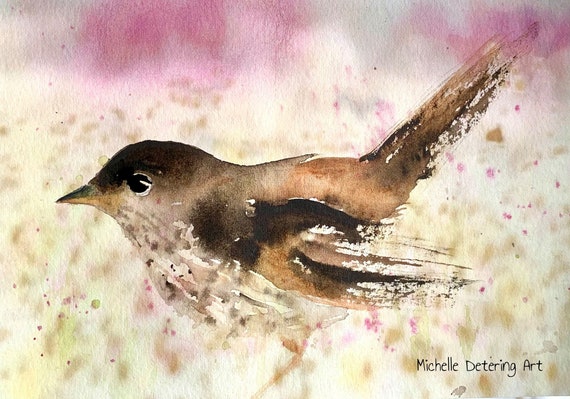This is a detailed watercolor painting by Michelle Dettering, as indicated by the black print in the bottom right corner. The focal point is a small, predominantly brown bird facing to the left. The bird's chest is white with brown specks, and the tips of its wings are white. It has a distinctive black eye visible from the side view. The background features an abstract mix of white, green, and pink areas, with dots and blurs creating a sense of depth. Further in the distance, there are subtle, blurry images of pink and white, contributing to the soft, ethereal feel of the painting. The background shades smoothly from ivory to delicate pink hues at the top and bottom, complementing the bird's subtle coloration.